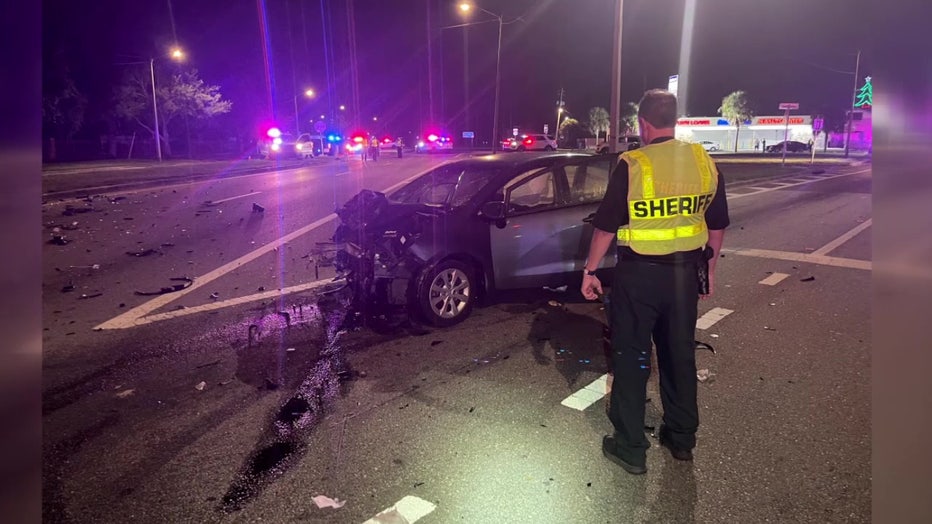The photo captures a devastating nighttime car crash scene at a busy intersection. Dominating the center is a gray compact car, with its front end completely obliterated, scattering debris across three lanes of the road. The car's airbags are deployed, and the driver's door swings open, revealing an empty seat. Illuminated by flashing blue and red police lights emanating from multiple patrol vehicles in the background, the scene is chaotic yet starkly detailed. 

A man stands in front of the wreck, identifiable as a sheriff by his yellow vest with "Sheriff" emblazoned on it. He is dressed in black attire, complete with a short-sleeve shirt, pants, boots, a watch on his left wrist, and a pistol holster on his right hip. His short hair and the gravitas of his stance add to the tension of the moment. Nearby, street lamps cast additional light on the scene, while distant buildings and a gas station can be seen on the right, contributing to the urban landscape. Tree silhouettes and a Christmas tree decoration form part of the background, highlighting the season. The street's oil spills glisten under the artificial lights, accentuating the grim reality of the accident.